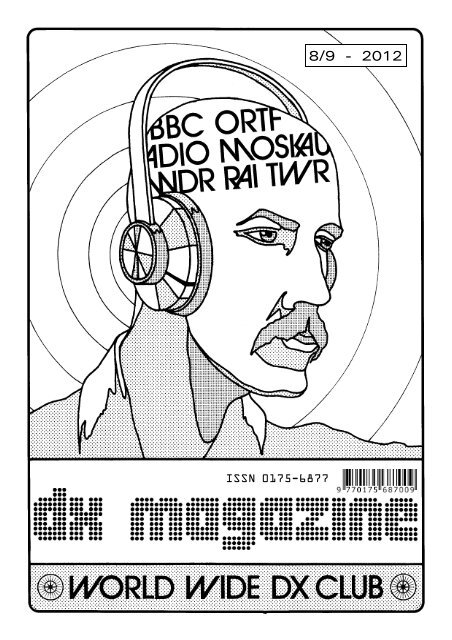The image appears to be a black and white, digitally animated magazine cover, dated August 9, 2012, with the text "A4-Line-2012" on the top right. Centrally featured, there is a black and white outline of a bald man’s head, neck, and left shoulder. The man is wearing over-the-head earphones, which are notably not connected at the top and extend outwards. He has grey eyebrows and a grey mustache but no beard. On his forehead, three lines of text can be seen: "BBC ORTF," "Radio MOSKAU," and "NDRAITWR." Swirling black patterns decorate the white background. At the bottom, the text reads "DX MAGAZINE," followed by "WORLDWIDE DX CLUB." Additionally, there is the serial number ISSN 0175-6877-DX-MAGAZINE-9770-175-687-009_PLATFORM.